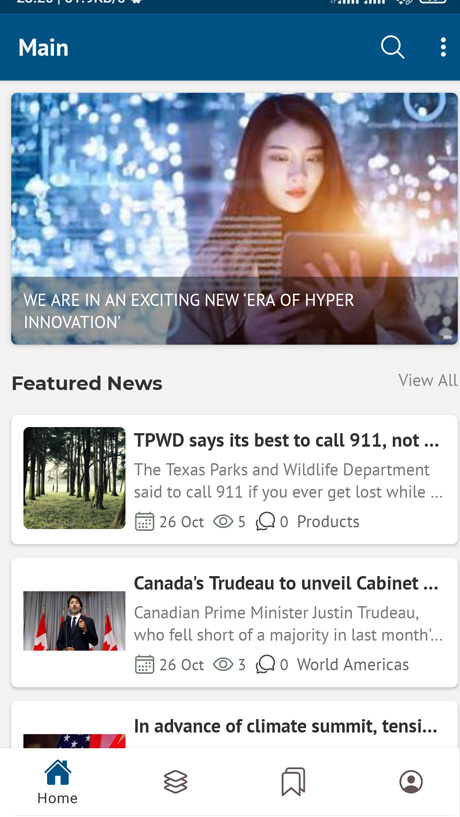This image is a screenshot of a mobile webpage. At the top, there's a prominent blue stripe featuring the word "Main" on the left-hand side, along with a search icon and a hamburger menu on the right-hand side. Just below this stripe, there's an image of a woman standing in front of a glass window with raindrops, reflecting light in the background. She is looking intently at a tablet. A text overlay at the bottom of the image reads, "We are in an exciting new era of hyper-innovation."

Beneath the image, the page transitions to a white background featuring the "Featured News" section. The first news headline advises, "TPWD says it's best to call 9-1-1, not the Texas Parks and Wildlife Department, if you get lost in the woods." The second headline states, "Canada's Trudeau to unveil new cabinet." The third news item is cut off, starting with "In advance of climate summit," followed by the incomplete phrase, "tension."